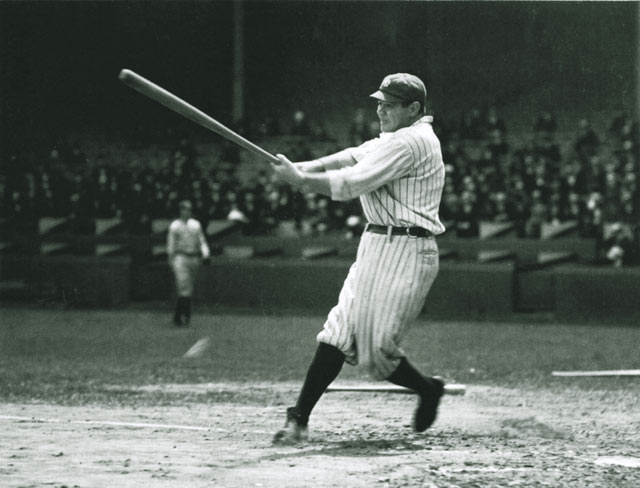This is a vintage black and white photograph capturing a historic moment on a dirt baseball field. The central figure, possibly Babe Ruth, is mid-swing, facing left and suggesting a powerful left-handed hit. He is clad in a white uniform adorned with darker pinstripes, a dark cap, and black knee-high socks, with his right foot kicked up, toe pointed to the ground. The action unfolds against a backdrop of a partially filled stadium, with visible spectators engrossed in the game. Behind the batter, an umpire stands near the edge of the field, and to the left, another baseball player in a similar uniform can be seen walking. The scene exudes a timeless atmosphere, capturing the dynamic energy of early baseball.